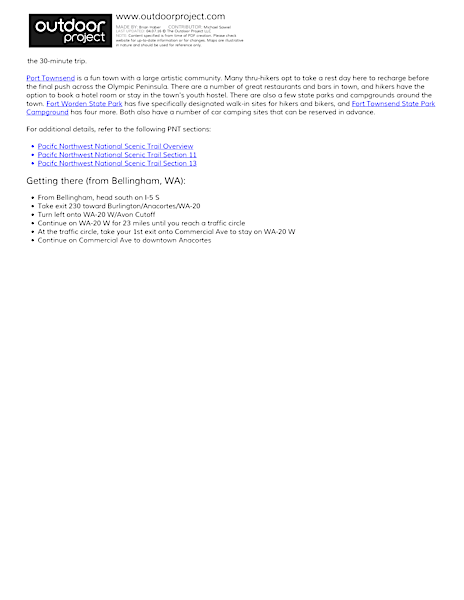This is a detailed screenshot of information presented on a white background with black text and several blue hyperlinks in the upper left corner. A black rectangle with white font contains the title "Outdoor Project." To its right, the URL "www.outdoorproject.com" is displayed. Below the black rectangle, there is a detailed paragraph which starts with, "Port Townsend is a fun town with a large artistic community." The text explains that many long-distance hikers choose to take a rest day here to recharge before continuing their journey across the Olympic Peninsula. The description highlights the town's numerous restaurants, bars, hotels, and a youth hostel. Additionally, it mentions several nearby state parks and campgrounds, including Fort Worden State Park, which offers five walk-in sites for hikers and bikers, and Fort Townsend State Park campground, with four more designated sites. Both parks also provide car camping sites that can be reserved in advance. The passage concludes with a reference to more information available in the "P and T" sections.